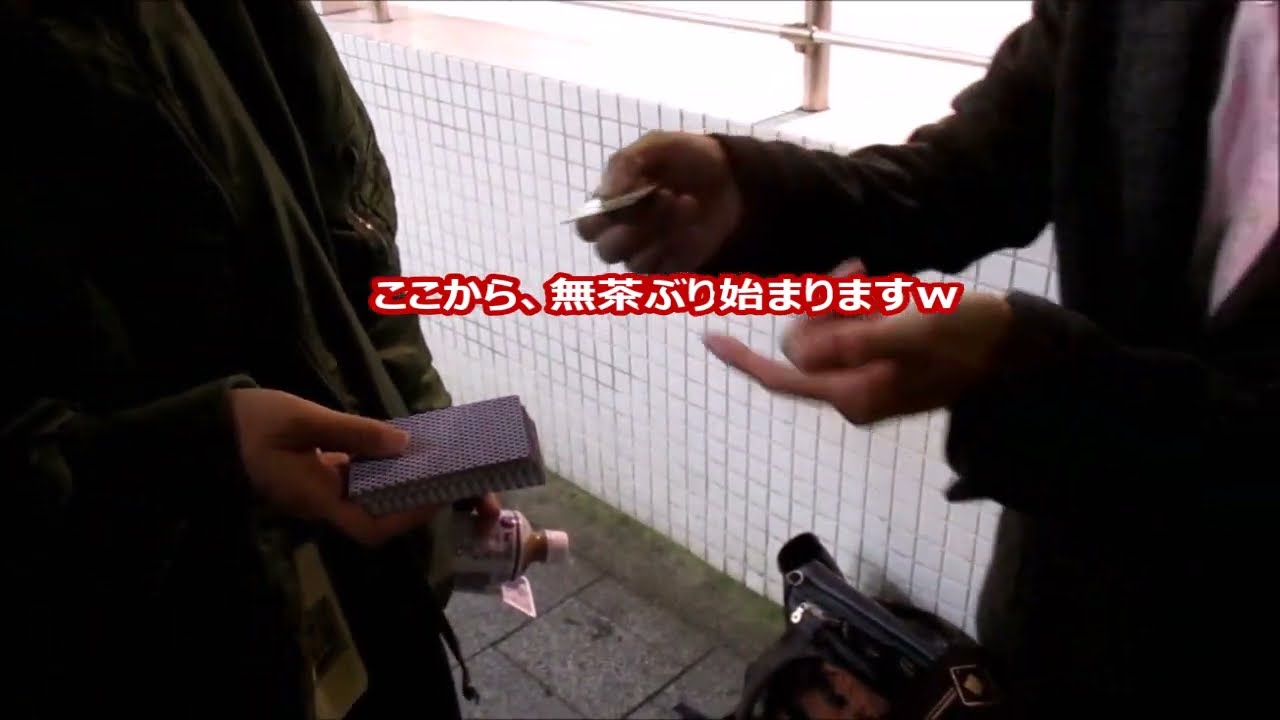The image depicts a person sitting cross-legged on a tan carpet, facing the viewer but only visible from around the mid-torso down. The individual is adorned in a navy sweat jacket with gold stripes on the sleeves and gray shorts, indicating a comfortable, casual setting. The person's hands rest on a vibrant lime green cloth that covers a small table, on which lie two black and white printed pieces of paper or pamphlets. To the right of the person, near their knee, one can spot a black pen and a remote control. Additionally, there is a wooden baseboard on the left side against the wall, which features grayish-bluish wallpaper. The photograph is overlaid with white text in an Asian language, possibly Korean or Chinese, featuring characters with a distinctive purple drop shadow, offering some form of explanation or advertisement.